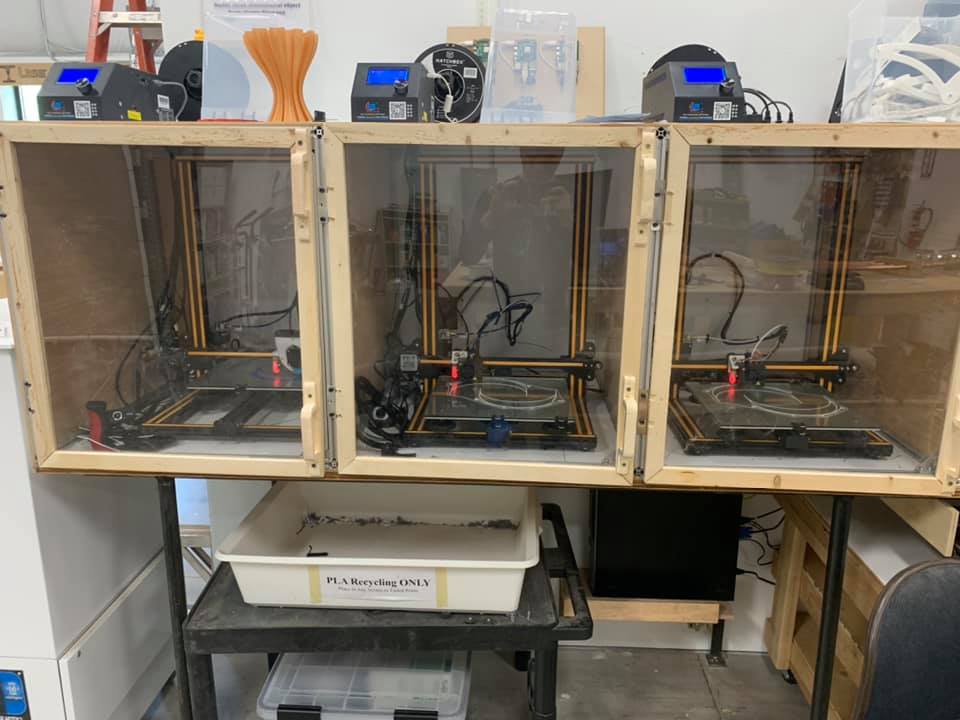This image captures a home workshop or possibly a small company workshop with a distinct DIY feel. Dominating the scene are three wooden cabinets that are segmented into separate workstations, each encased with plexiglass doors on two sides and wooden walls on the other. Inside these cabinets sit three 3D printers, characterized by their flat metallic bases, complex wiring, and sliding bars which are visible. Each printer is squared, featuring a gray inset plate, and has an upper plate with gold trim and a prominent red unit at the back of each one. 

Prominently atop these cabinets, various electronic components, including black cube-like units equipped with blue LED screens, are neatly arranged, presumably as part of the organizational structure or for additional storage. The open space beneath the printers houses a black metal cart on wheels, topped with a white bin clearly labeled 'PLA Recycling Only,' indicating a specialized function for recycling 3D printing materials; another bin sits below it.

Despite apparent confusion over specific details in the captions, the image clearly shows a well-arranged mini-lab dedicated to 3D printing, equipped for efficient recycling and possibly other auxiliary tasks.